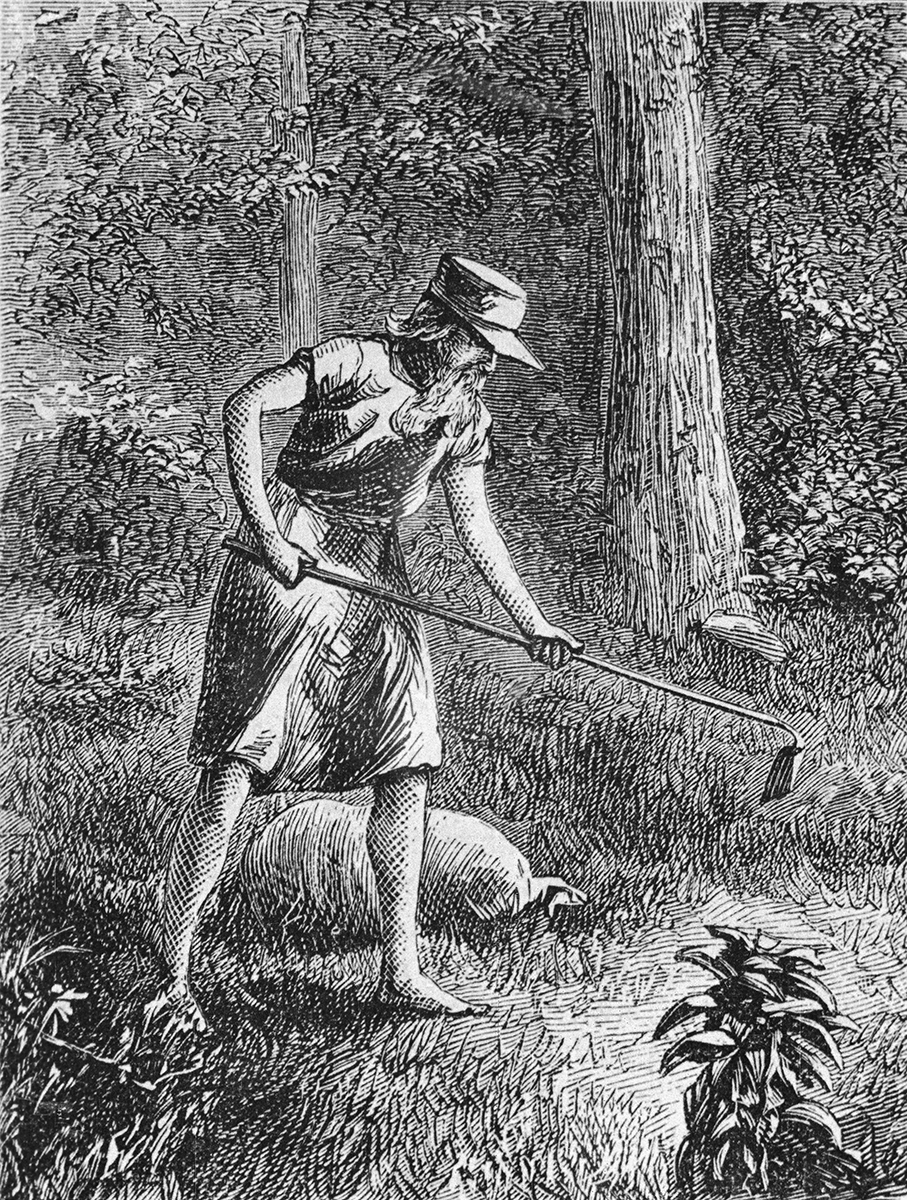This black and white sketch is a highly detailed drawing that depicts a man tilling the soil in a forested area. The man, who appears to be from an earlier time period, is dressed in a tunic-like garment that flows down to his knees. He also wears a short-sleeved top and perhaps some form of tights, as his bare legs are not visible. Notably, he is barefoot. On his head is a distinctive hat with a flat rectangular flap. The man has long hair that reaches his shoulders and a very long beard that extends to the middle of his chest. He is using a gardening tool, specifically a hoe with a long metal handle and a flat, wide end, which he holds while leaning towards the ground. Surrounding the man are tall trees with varying trunk widths, as well as bushes and other plants, all meticulously shaded to highlight the depth and texture of the forest environment.